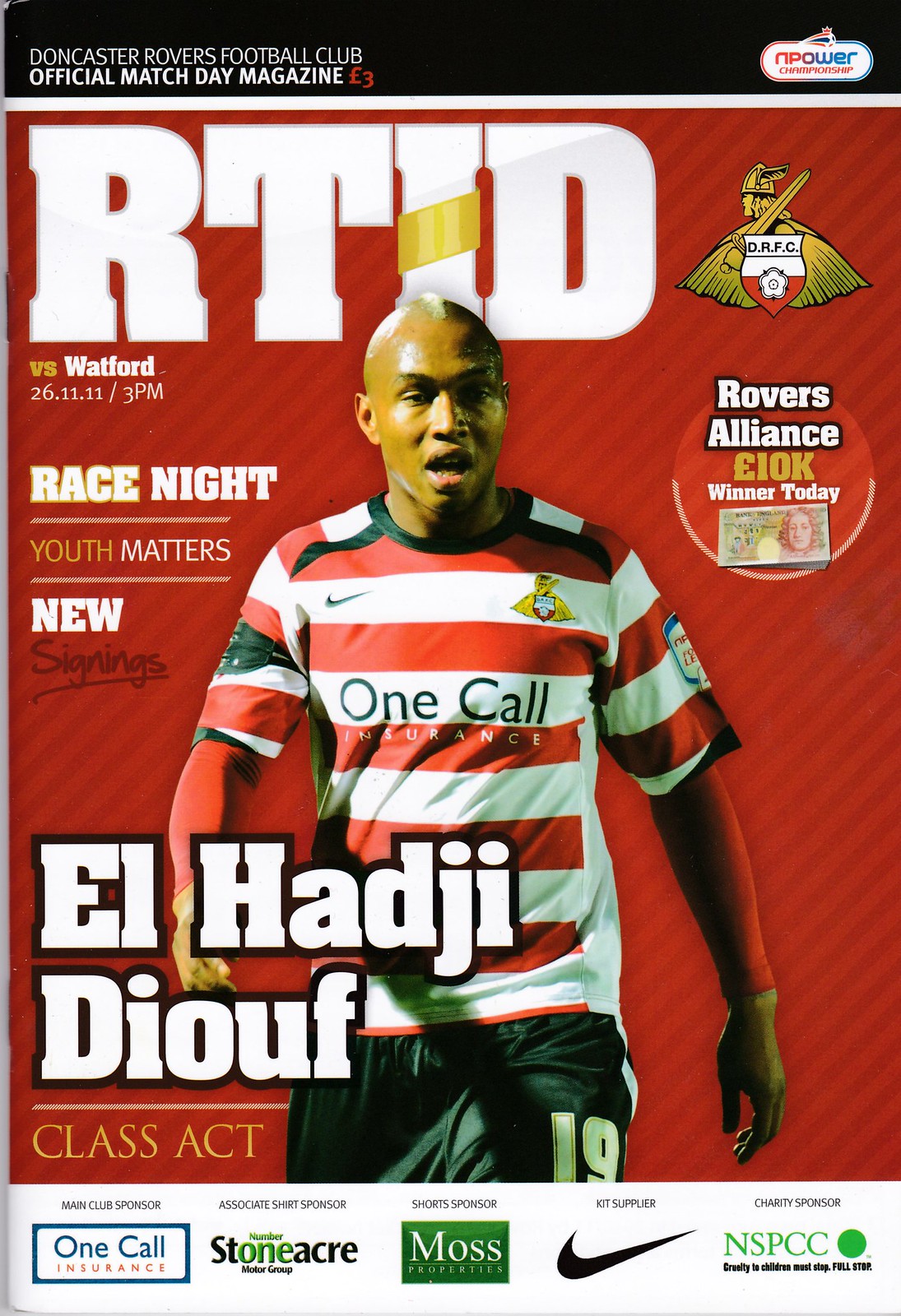This image is a highly detailed scan of the front cover of a football program, likely the Official Match Day Magazine for Doncaster Rovers Football Club. The cover is dominated by a striking design featuring diagonal stripes in various shades of red. A black header at the top declares "Doncaster Rovers Football Club Official Match Day Magazine" in white print. The right side of this header displays the NPower Championship logo, characterized by its red and blue submarine shape, and the price "£3" in red.

Prominently displayed in large, bold white letters across the red background is "RTID," with the Doncaster Rovers Football Club (DRFC) crest to its right— a gold Viking with a sword and a red-and-white shield. Below this is the match information: "Versus Watford 26.11.11 / 3 PM", followed by other key elements such as "Race Night," "Youth Matters," and "New Signings."

The central image showcases a dark-skinned man, identified as El Hadji Diouf, an athlete wearing a red-and-white striped jersey paired with black shorts adorned with the number 19. The jersey is sponsored by One Call Insurance. The player's name appears bold in white text on the lower left, accompanied by the phrase "Class Act" in elegant gold print. 

Rounding off the key visual elements, there is a red circle with white print and black outline on the right that reads "Rovers Alliance," emphasizing a "10K Winner Today." At the bottom, the program features a white footer listing various sponsors: One Call Insurance as the main club sponsor, Stoneacre Motor Group as an associate shirt sponsor, Moss Properties as an insurance sponsor, Nike as the kit supplier, and NSPCC with its compelling child protection tagline.

Overall, the design utilizes a primary color scheme of red, white, black, and accents of gold, creating a visually captivating cover brimming with information and club pride.